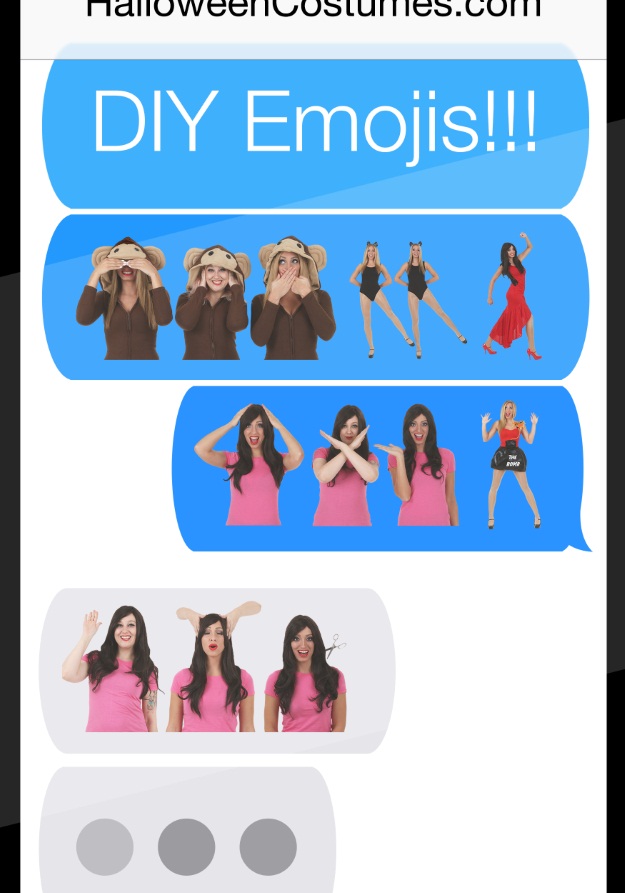This image, designed to resemble a mobile phone screen with a white background and a black border, appears to be a mock-up advertisement or social media post from HalloweenCostumes.com. At the top of the screen, partially visible text reads "Halloween Costumes dot com," suggesting the source of the advertisement. The central feature is a simulated text conversation under the headline "DIY emojis!!!" which showcases various do-it-yourself emoji costume ideas.

In the first text bubble, a woman dressed in a monkey costume performs the "see no evil, hear no evil, speak no evil" poses, wearing either a black or brown sweater with a monkey hat. Following this, there are emojis of twin women in black leotards and high heels, dancing with their legs out, and a woman in a red cocktail dress dancing. Below this, another text bubble displays more emoji-inspired costumes: a woman in a pink shirt demonstrates three different expressions, one with her hands on her head in surprise, another forming an 'X' with her hands, and the last with her hand out to the side, smiling. Accompanying this, there is a woman in a skirt with "time bomb" written on it, imitating a bomb about to explode with a surprised expression.

Lastly, the next text bubble shows a woman dressed in a pink shirt with long hair, portraying three distinct emojis: one waving, another appearing to receive a head massage, and the third simulating a haircut with scissors next to her hair. Three dots underneath indicate that another message is about to be sent, enhancing the text message effect of the image.